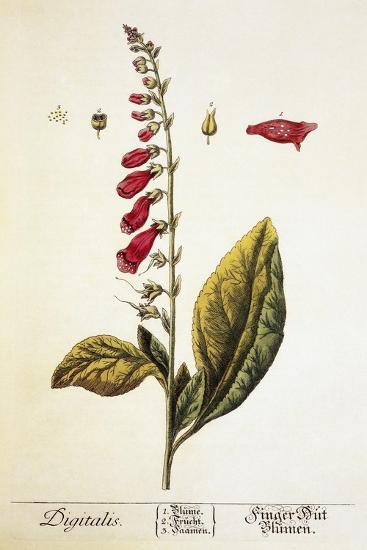The image is a detailed, vintage botanical drawing of the plant Digitalis. Positioned prominently in the center, the plant features large green leaves at the base with smaller leaves interspersed among the stalk. As you move up the stalk, you see a series of red bell-shaped flowers that diminish in size. The drawing illustrates different parts of the plant, including an enlarged image of the seed on the upper left and the bud on the upper right. The colors used are dark reds, dark greens, and gold highlights, giving the image an antique feel typical of a botanical directory or guide. At the bottom left, the name "Digitalis" is written in script, and nearby, possibly in German, are the words "finger blooming." Additionally, there is text featuring the numbers 1, 2, and 3, likely indicating various parts of the plant, along with more cursive text on the lower right, creating a sophisticated, filigree touch.